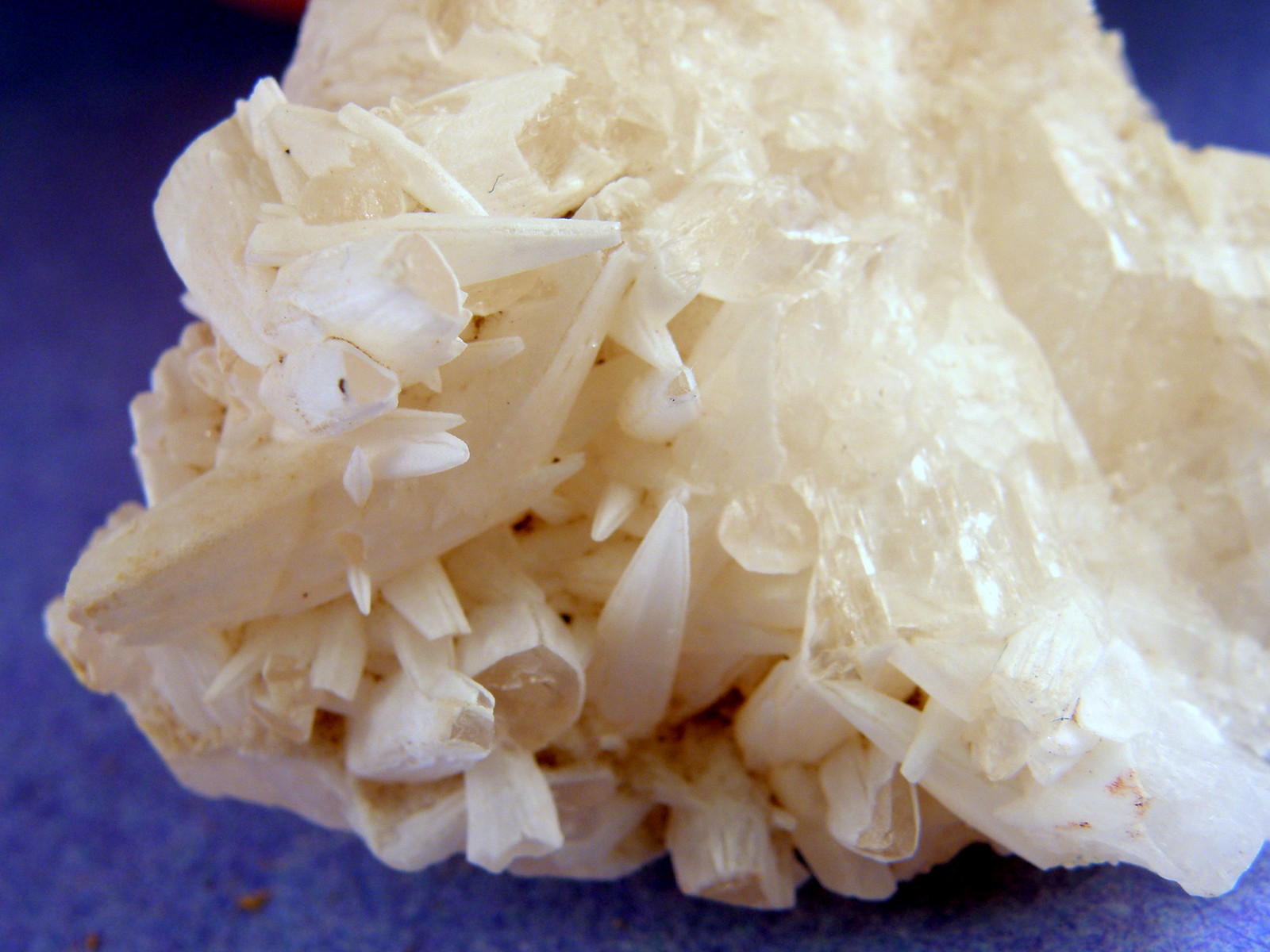The close-up image showcases a unique rock resting on an unidentified medium blue surface. The left side of the rock displays a light brown to cream color and features an unusual texture reminiscent of small beach shells fused together. This side is jagged, with numerous pointed edges jutting out unpredictably. In contrast, the right side of the rock exhibits characteristics similar to quartz, with predictable, sharp edges indicative of crystallized formations. The juxtaposition of the rock's two distinct sides creates an intriguing natural composition.